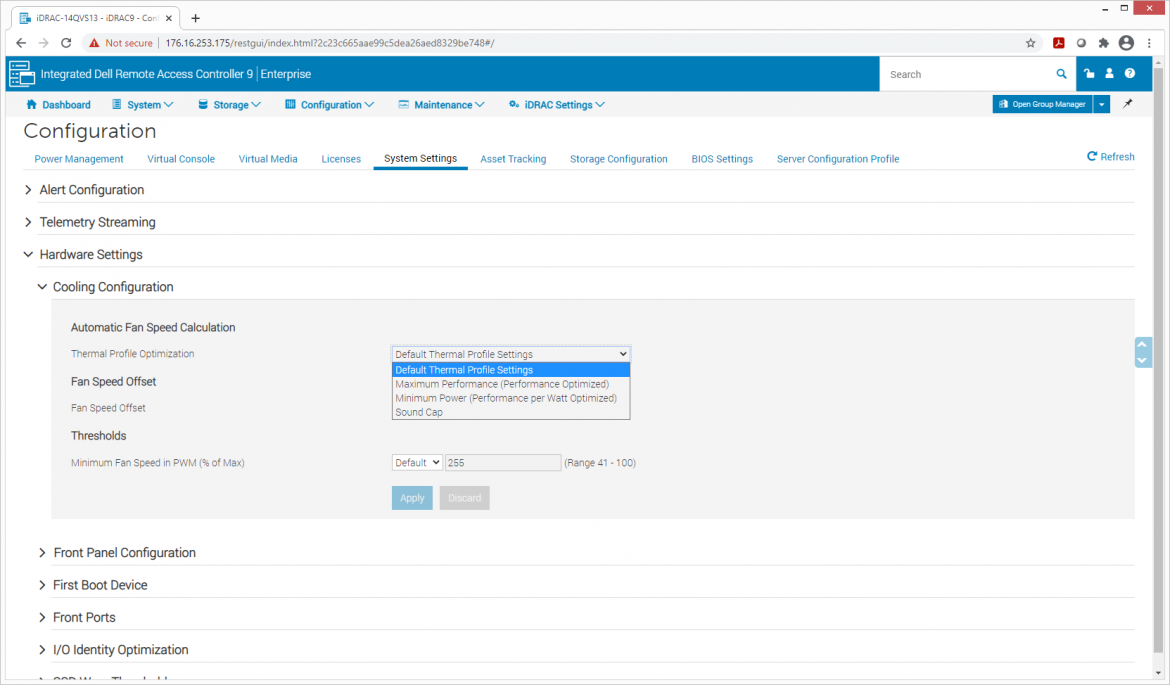This screenshot displays a detailed interface of the Integrated Dell Remote Access Controller 9 (iDRAC9) Enterprise dashboard, likely from Dell Technologies. The header prominently identifies the application, and below it lies a blue navigational menu with several options: Dashboard, System, Storage, Configuration, Maintenance, and iDRAC Settings. The main content area features a white background with a section titled "Configuration," presenting a list of sub-menus in gray: Alert Configuration, Telemetry Streaming, Hardware Settings, and Cookie Configuration. Additionally, there's a light gray rectangle stretching horizontally across the screen, containing settings related to automatic fan speed calculation, such as Fan Speed Offset and Thresholds.